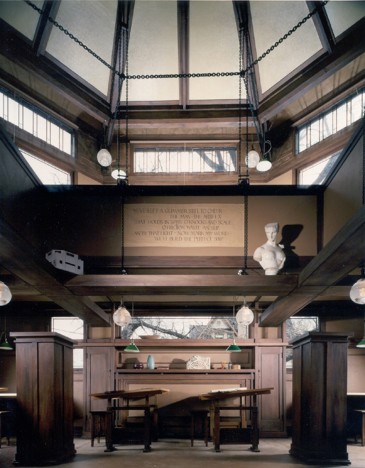The image depicts the interior of a grand room with tall, white windows extending from the floor to the high ceiling, which narrows into a conical or pyramid-like shape adorned with light beige paneling. The walls are predominantly brown, composed of rich mahogany wood that lacks much grain. The room features wooden desks or pedestals, suggesting it could belong to a university lecture hall, a church sanctuary, or a museum's special collection section. There are benches and hanging light bulbs illuminating the space. A notable detail is the presence of a bust of a white male placed on a shelf, with an engraved plaque on the wall, although the text is unreadable. Additionally, windows reveal an overcast outdoor scene with visible trees, and there is a small floor-level window. A prominent arch with a chain across it further accentuates the room's architectural grandeur.